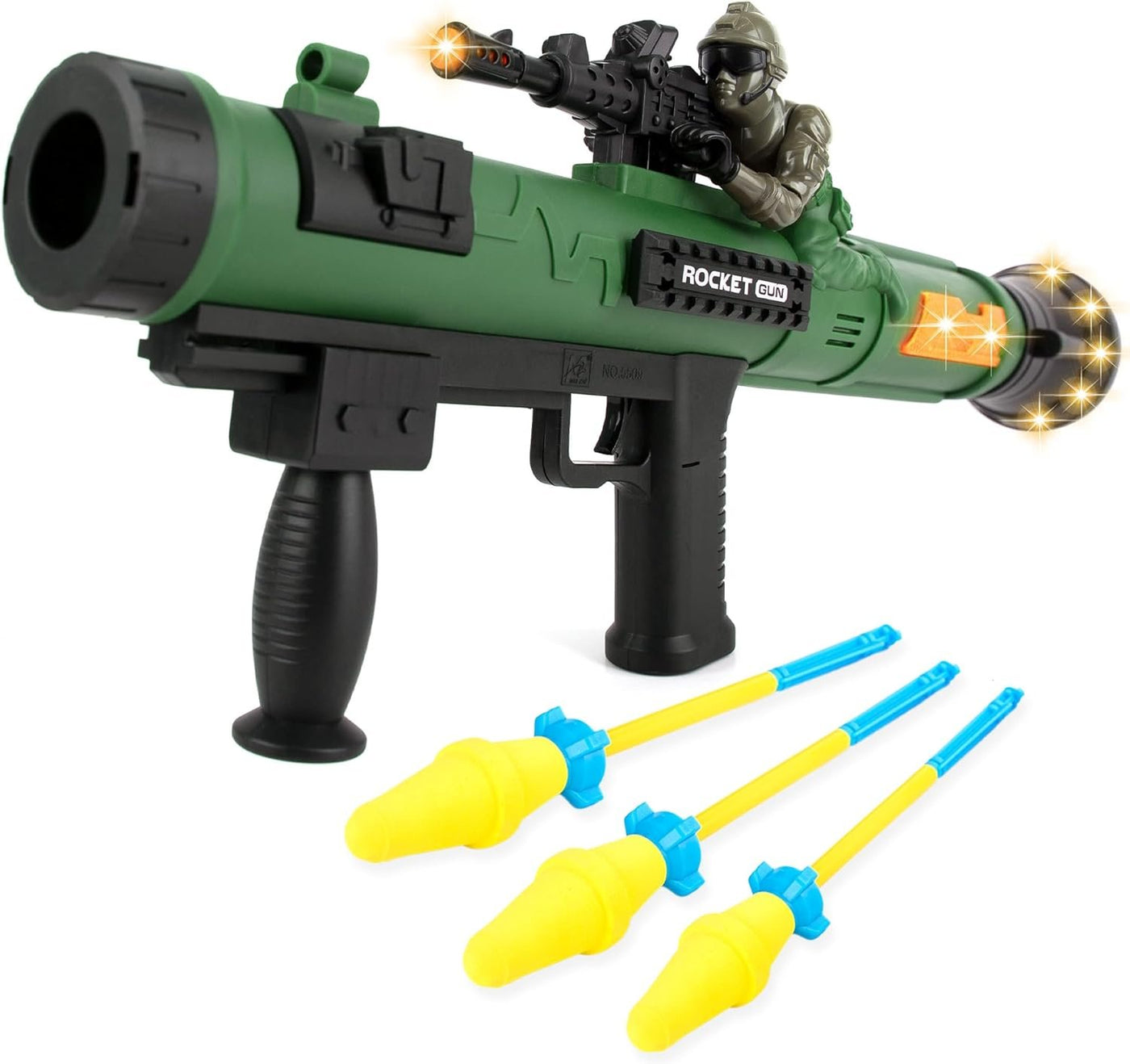The image depicts a detailed toy rocket facing to the left. The firing end of the rocket, located on the left side, features a black ring surrounding it. The main body of the rocket is predominantly green with a small, black-shelled scope situated near its tip. This holder adds to the intricate design.

The rocket's handles and rail, both utilized for gripping, are centrally located and also colored in black, continuing this theme towards the front end, near the firing mechanism. The rear of the rocket, where the exhaust expels, showcases a combination of black accents and yellow lights with an additional orange piece attached.

Mounted on top of the rocket is a toy soldier. The soldier’s attire features pants that match the green hue of the rocket's body, while the upper half is a grayish-green color. The soldier is depicted in the action of firing a machine gun.

To the side and below the soldier, a label reads "rocket" and "gun" respectively. The word "rocket" is in white, encased by a black bar, and "gun" is in black within a white box.

Adjacent to the main rocket on the white background lies a set of three smaller toy rockets. These mini rockets are characterized by yellow tips, blue holders, and handles that transition from yellow at the top to blue at the bottom.